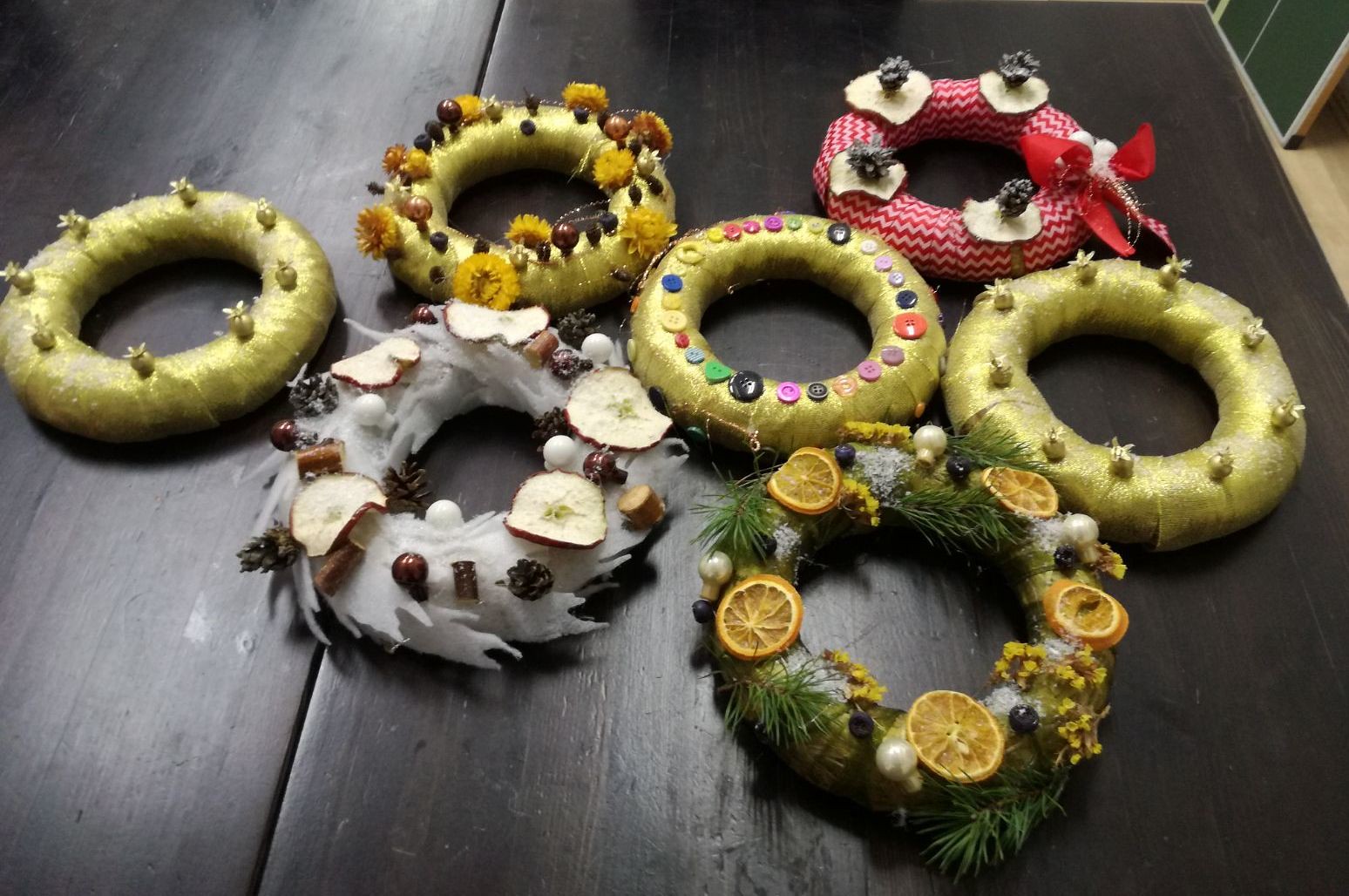This color photograph captures an assortment of intricately decorated small wreaths, each about the size and shape of donuts, meticulously arranged on a darkly painted wood table. To the right emerges a green-surfaced turned-up table with a white rectangular border, resting on a tan-colored floor. 

There are seven wreaths, each uniquely embellished. The first wreath on the left is adorned with small gold apples and leaves. The second features a mix of yellow dandelions, small black, maroon, and pink circles. The third wreath stands out with a diverse array of colored buttons, including black, green, light gray, red, beige, yellow, dark blue, olive, and more. Similar to the first, the fourth wreath is lined with golden apples.

The fifth wreath is white, embellished with hard-to-identify cut fruit, brown circles, pieces of wood, and pine cone-like elements. Next, another white wreath is decorated with orange peels, dandelions, small black circles, pearl-like mushrooms, and dark green evergreen leaves. The final wreath boasts a red patterned cloth with white zigzag designs, a red bow accented with white puff balls, gold ribbon, pine cone-like pieces, and unidentified circular white elements on top.

This assembly suggests a dedicated effort in creating homemade, artistically-varied wreaths, each contributing to a rich tapestry of textures and colors against the dark wood tabletop backdrop.